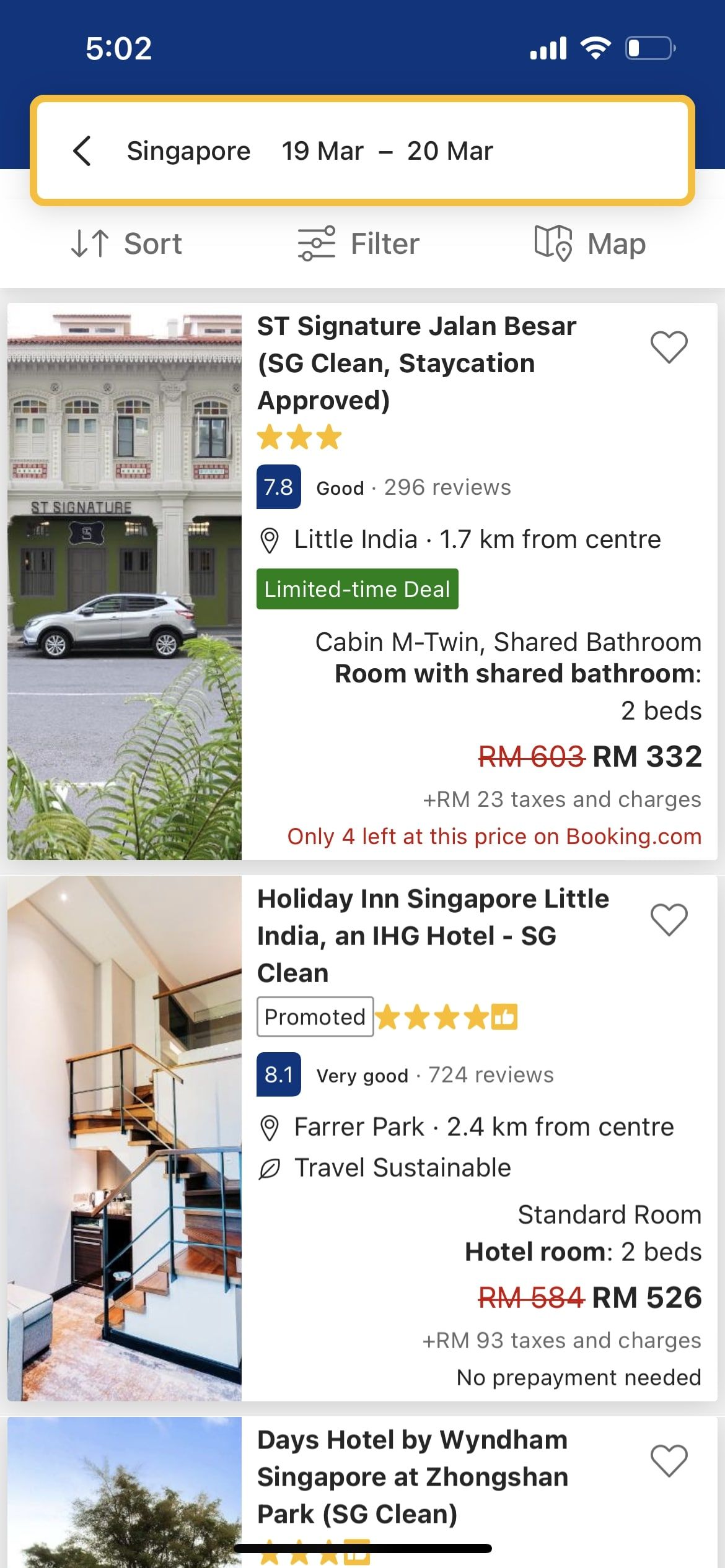This image depicts a smartphone screen with a blue background. The time "5:02" in white font is displayed in the top left corner, with icons for Wi-Fi and battery life to the right, indicating a low battery. Below these, a yellow square with a white background features a black arrow pointing left and text that reads "Singapore, 19 Mar - 20 Mar."

Underneath this information, a menu appears on a white background with gray font. The menu includes icons for sorting (denoted by up and down arrows), filtering (three lines with circles), and a map (labeled "map" with a map icon).

The first listing has a gray square outline and shows a photo of a building, a silver 4x4 vehicle in front, green bushes, and a gray road. To the right of the image, the text reads "ST Signature Jalan BCR, SG Clean Staycation Approved" with a gray heart icon next to it. Below this, there are three yellow stars and a 7.8 rating in a blue square with white font. Text in black on a white background reads "Good, 296 reviews." Additional information below indicates "Little India, 1.7 kilometers from center," with a limited time deal displayed in a green square with white font.

The room type listed is a "Cabin M-Twin, shared bathroom, room with shared bathroom, two beds." The original price of RM603 is crossed out in red, with a discounted price of RM332 in black. Additional charges include "+ RM23 taxes and charges." The text in red warns, "Only four left at this price on booking.com."

A gray line separates listings, leading to another image of stairs and a white wall. Beside this is the text for "Holiday Inn Singapore Little India, an IHG Hotel - SG Clean," followed by a gray heart icon. An adjoining gray box with gray lettering notes this is a promoted listing. The rating is denoted by four yellow stars within a yellow box and a white thumbs-up icon. Below, the rating of "8.1" is displayed in a blue box with white font, followed by "Very Good, 724 reviews" in gray font on a white background.

Further details show it is "2.4 kilometers from center" and mentions "Travel Sustainability." The room type is listed as a "Standard Room, Hotel Room, two beds" with the original price of RM584 crossed out in red, and a discounted price of RM526 in black. Additional costs include "+ RM93 taxes and charges" with a note stating "No prepayment needed."

Another gray line separates this listing from a mention of "Days Hotel by Wyndham Singapore at Zhongshan Park, SG Clean." The name is crossed out in black, and three stars along with a thumbs-up icon are followed by a gray heart. The accompanying image shows a blue sky and some green trees.